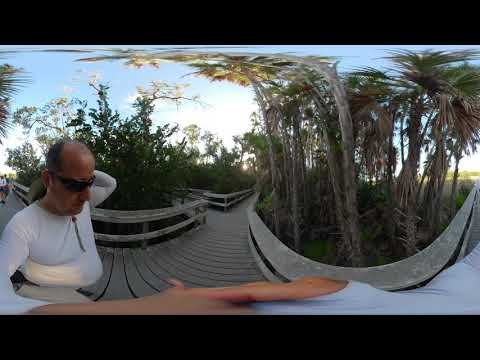The photograph captures a slightly surreal scene, created by the distortions of a convex or concave lens. Central to the image is a man in the foreground, positioned towards the left side. He is wearing a white, long-sleeve shirt with a zipper down the middle and dark black sunglasses. His bald head has a bit of hair above his ears. His left hand is behind his head, possibly scratching it, and his right hand reaches towards the front of the camera, adding to the distortion effect.

The setting is an outdoor wooden boardwalk, evidently part of a park or nature preserve. The boardwalk meanders in multiple curvy paths, bordered by fencing. The area is flanked by a variety of trees and bushes, including distinctive palm trees. Behind the walkway, the sky suggests a mix of blue and light, hinting at a late afternoon with the sun preparing to set. The bright sunlight filtering through the clouds adds to the whimsical, slightly skewed perspective of the photograph.